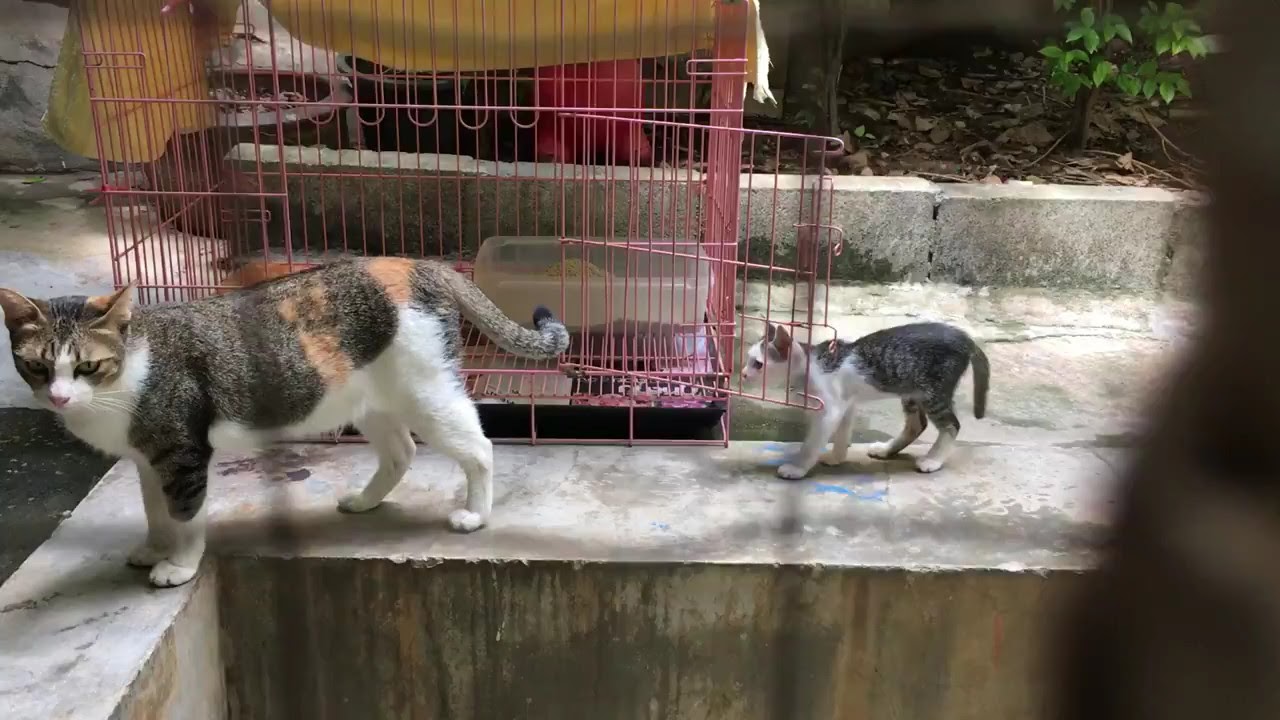In this high-resolution outdoor image taken during daylight, a wide rectangular scene is observed from behind a gate, marked by two faint vertical gray lines. The focus is on a concrete raised foundation where multiple cats are perched. Prominently, there is a large Torby cat on the left, featuring a blend of calico colors—orange, white, and shades of brown with tabby markings, yellow eyes, and a pink nose. Behind the Torby is a smaller kitten with similar fur colors. In front of them sits a notable large pink cage containing a sheer plastic litter box at the back right corner. The cage also has a yellow fabric draped on top, partially cut off at the image's top edge. The background reveals more concrete slabs, scattered leaves, rocks, sticks, and a vine with green foliage amidst a brush-filled area. The image is bright, clear, and free of any text or numbers.